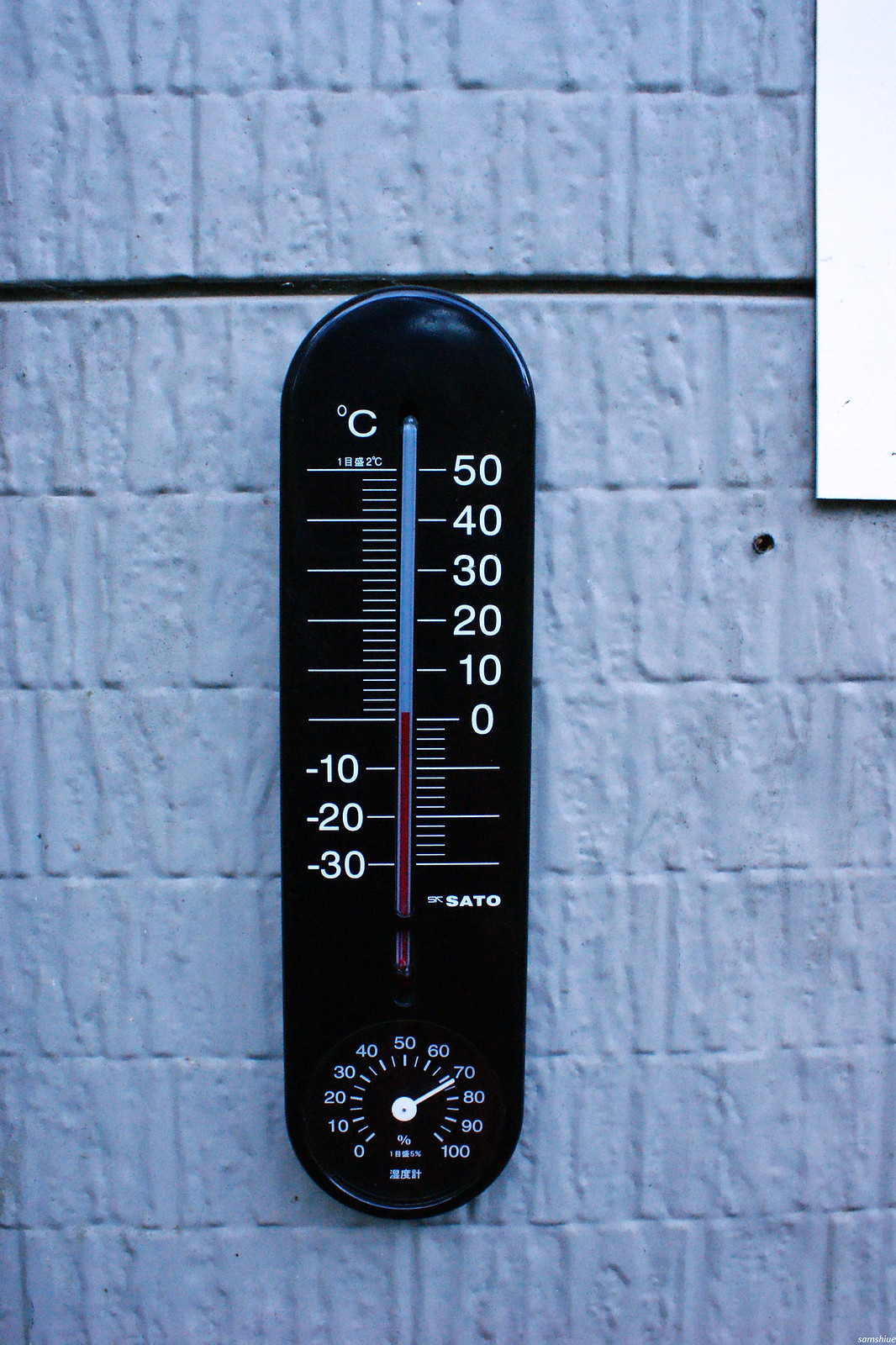This image showcases a sleek, modern outdoor thermometer mounted against a light blue or white wall. The thermometer, primarily black with a pill-shaped design, measures temperature in Celsius. The red mercury indicates a current temperature of 0°C. 

The thermometer is meticulously detailed, featuring tick marks on both sides. The left side of the thermometer displays negative values, marked at -10°C, -20°C, and -30°C, while the right side shows positive values, rising in increments of 10 up to 50°C. A blue background color is visible where the mercury is absent. At the top left side of the device, a white "C" denotes the Celsius measurement.

The base of the thermometer includes a circular, odometer-like dial with a pointer that extends to the 70 mark. This dial might represent an additional metric, perhaps Fahrenheit, though it isn't clearly indicated. The dial is marked in increments of 10, ranging from 0 to 100, accompanied by a percentage sign and some other unreadable characters, adding to its multifunctional appearance. The overall design and detailing emphasize its modernity and functionality.